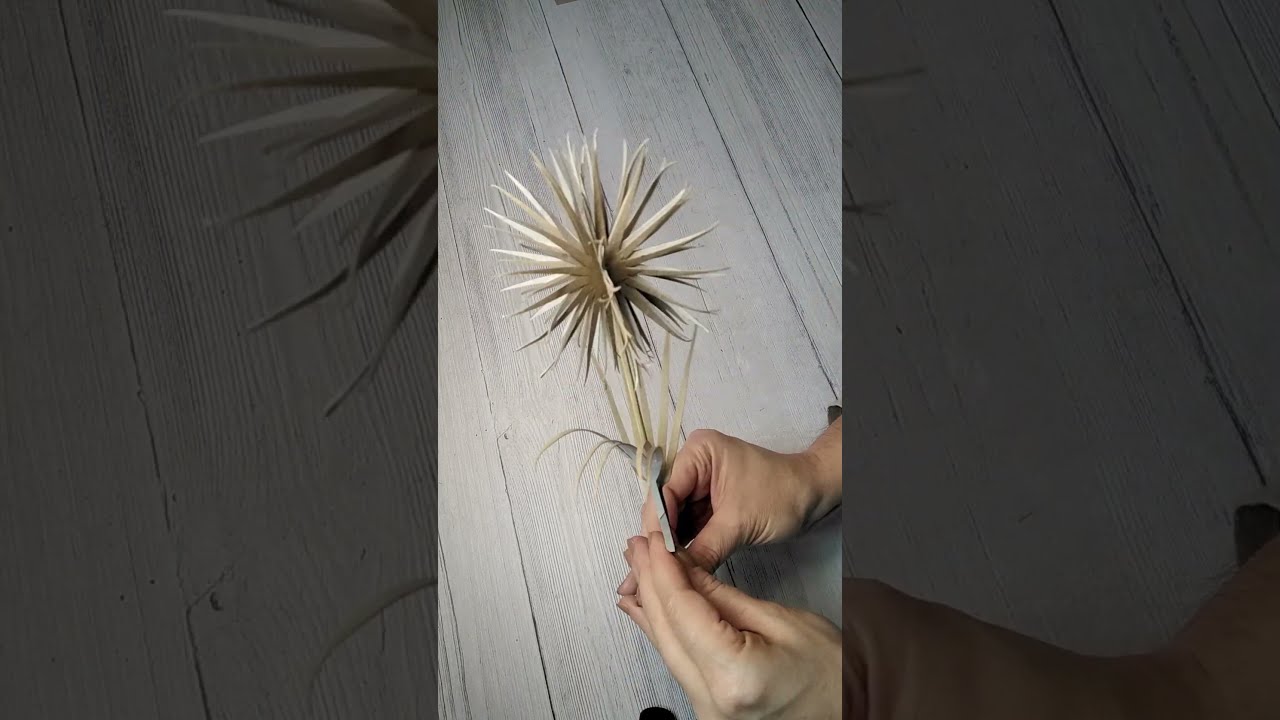In the center of the image, two Caucasian hands are holding a paper-crafted flower, characterized by its long, straight, light tan cardboard stem and thin, pointy triangular leaves. The flower's top features a large, spiky, spherical bulb, with numerous long strips of the same cardboard material radiating outward, reminiscent of an opened milkweed pod. The entire scene is set against a light gray wood plank floor, which has been darkened and enlarged to create a textured background on both the left and right sides of the composition. The image is in portrait orientation, emphasizing the craftsmanship and unique texture of the paper flower.